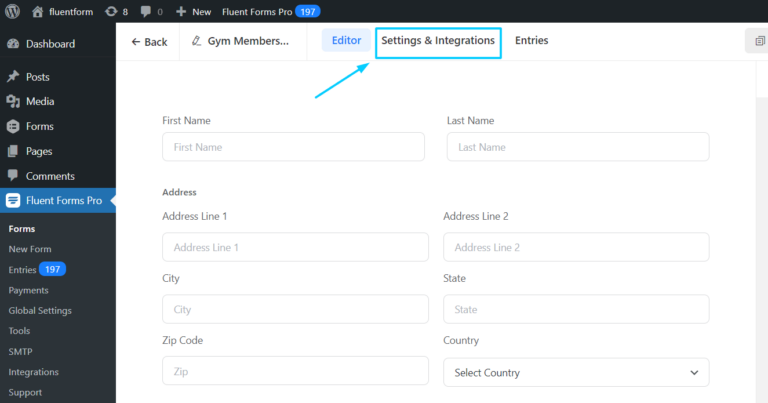The screenshot displays a web interface with a white background, featuring various icons and text elements. Across the top, there are several icons including a "W," a house symbol, "Fluent Form," a refresh symbol accompanied by the number 8, and a chat icon with the number 0. Additionally, there's a "Plus New" button and a "Fluent Forms Pro" label. 

To the left of the screen, there's a sidebar menu with multiple options such as Dashboard, Posts, Media, Forms, Pages, Comments, and Fluent Forms Pro, with the latter being highlighted in blue and accompanied by a blue circle bearing the number 197 in white. Below these options, sub-options include Forms, New Form Entries (also highlighted in blue and next to a similar blue circle displaying 197), Payments, Global Settings, Tools, SMTP, Integration Support, and "Gym Members" with the editor also highlighted in blue.

In the main section of the screen, labeled "Settings and Integrations" (encased in a blue rectangle with a blue arrow pointing towards it), there is a form layout including fields for "Entries," "First Name" with an empty input box, "Last Name" with another empty box, "Address," "Address Line 1" with another box, "Address Line 2" still with a box, "City" with a box, "State" with a box, "Zip Code" with a box, and "Country" with the respective input box. To the right side of the form, there is a vertical gray scrollbar for navigation.